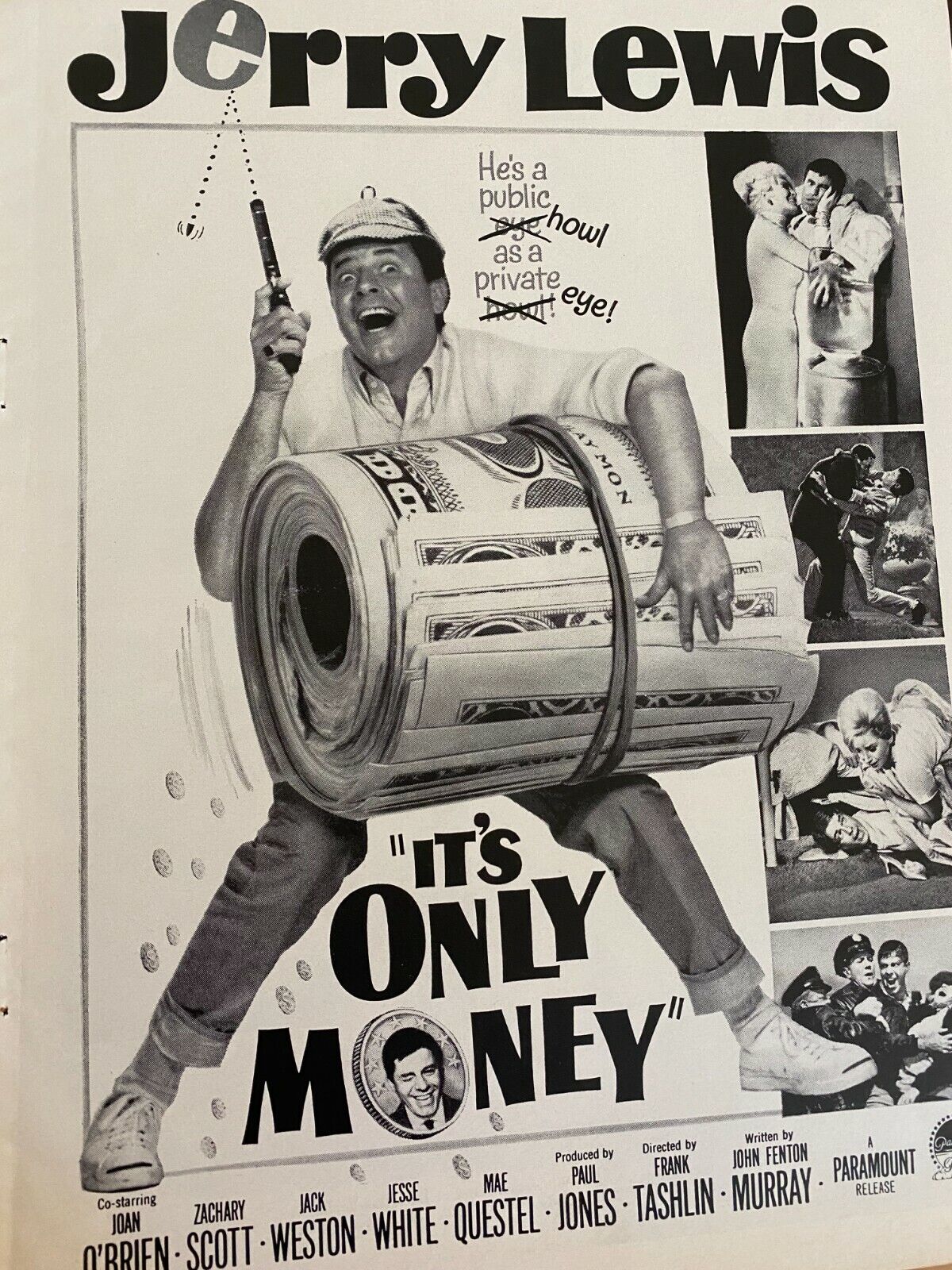The image is a vintage advertisement featuring Jerry Lewis prominently. At the very top, the name "Jerry" is highlighted, with a bullet seemingly fired from a gun in his right hand, striking and rebounding off the letter "E." Jerry Lewis is depicted holding an oversized bundle of one-dollar bills in his left hand, appearing to struggle under its weight. To the left of his head, there is text that reads "He's a public how or I," with the words "how" and "or I" crossed out, followed by "as a private" crossed out as well, leaving the phrase "He's a public I." To the right, the ad features additional images or illustrations, further enhancing the promotional material. The text "It's Only Money" is prominently displayed, likely the title of the advertisement or the context in which Jerry Lewis is being featured.